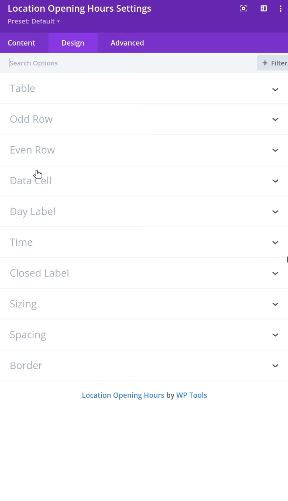This is a vertical image likely captured from a smartphone device, displaying a user interface with a predominantly white background. The interface appears to be from a settings or customization screen, characterized by its minimalistic design.

At the top of the screen, there is a purple rectangular header. In white text within this header, the following options are listed: "Location Opening Hours," "Setting," "Preset Default," "Content," "Design" (which is highlighted in a lighter shade of purple to indicate it is currently selected), and "Advanced."

On the upper right side of this header, there are three clickable icons for more information or options. Directly below this header, a gray search bar with the label "Search" is visible, accompanied by a "Filter" option on its right.

The interface includes a dropdown section beneath the search bar, featuring options such as "Table," "Odd Row," "Even Row," "Data Cell," "Day Label," "Time," "Closed Label," "Sizing," "Spacing," and "Border." Each option has a downward-pointing arrow next to it, indicating that they can be expanded for further customization.

At the bottom of the screen, in a pretty blue color, the text "Location Opening Hours by WP Tools" is displayed, indicating the tool or application being used.

This detailed and methodical layout suggests a user-friendly interface designed for easy customization of various settings related to location opening hours.